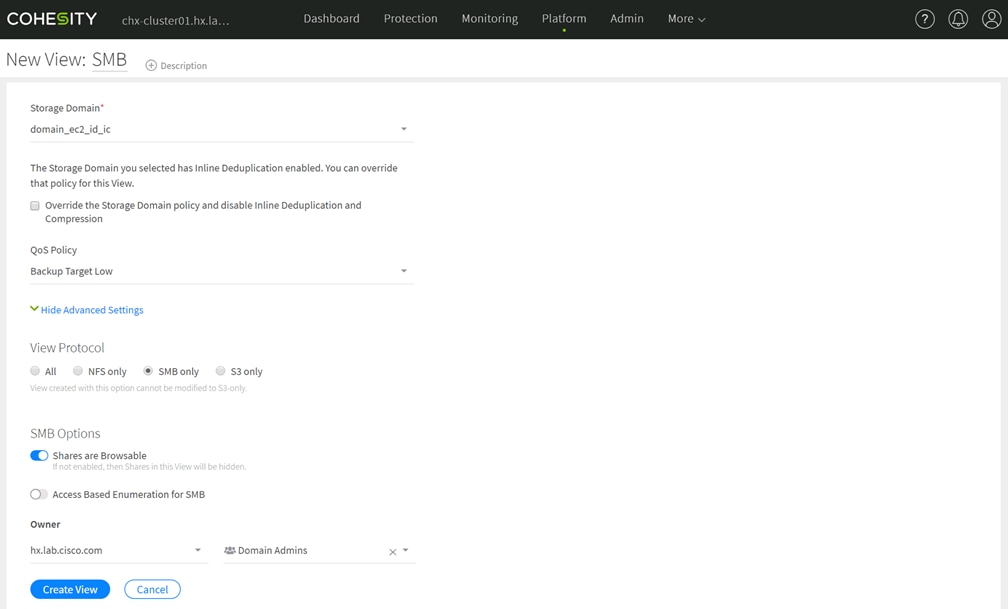The image showcases a Cohesity web interface. At the top of the screen, the Cohesity logo is prominently displayed, featuring an "S" designed to look like two green letter C's hooked together. This logo is situated within a black menu bar that contains the following menu options: Dashboard, Protection, Monitoring, Platform, Admin, and More, with a green dot highlighting the "Platform" section.

As you move down the interface, there is a section labeled "New View" with an "SMB" label next to it. A circular icon with a plus sign next to the label "Description" is visible. Below this, there is a mention of the "Storage Domain" with adjacent details about the domain. It states that the selected storage domain has inline deduplication enabled, with an option to override this policy for the current view. 

There is a gray button labeled "Override the Storage Domain Policy and Disable Inline Deduplication and Compression." Further down, there is an option to "Hide Advanced Settings," indicated by blue text. Additional settings reveal the "View Protocol" section, where there are "SMB Options." Within these options, "Shares are Browsable" is turned on, while "Access-Based Enumeration for SMB" is turned off.